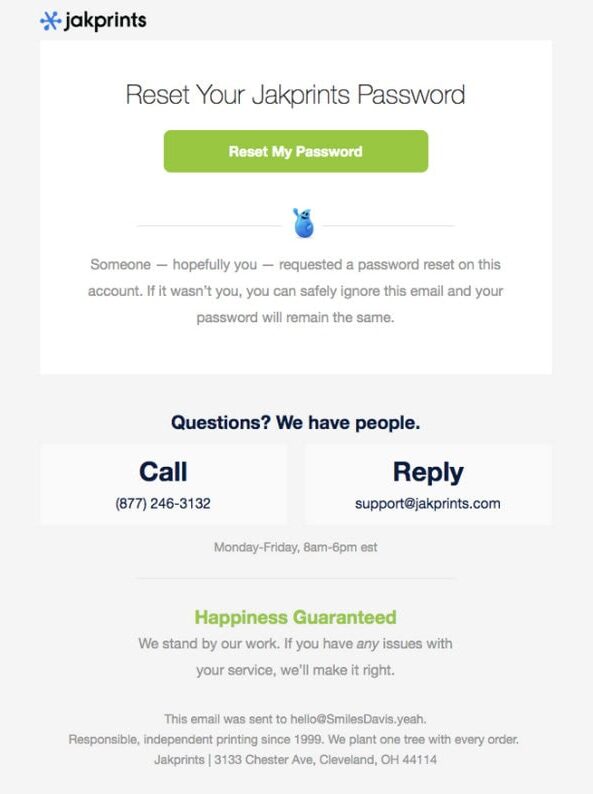In the image, the top section features a star icon beside the brand name "JackPrince." Below this, bold text reads, "Reset Your JackPrince Password." Centered prominently is a green button labeled, "Reset My Password." 

Immediately following, there's explanatory text stating, "Someone, hopefully you, requested a password reset on this account. If it wasn't you, you can safely ignore this email and your password will remain the same."

For further assistance, the image provides contact information: "Questions? We have people. Call 877-246-3132 or reply to support@jackprince.com. Our support hours are Monday to Friday, 8 AM to 6 PM Eastern."

A section of green text assures a "Happiness Guarantee," with a note that reads, "We stand by our work. If you have any issues with the service, we'll make it right."

The concluding part of the email includes details like the sender's email address, "hello@smilestavis," and company information: "Responsible, independent. Retained since 1999. We plant one tree with every order."

At the bottom, the company’s address is listed: "JackPrince | 3133 Chester Avenue, Cleveland, Ohio, 44114." The entire email is set against a plain white background.